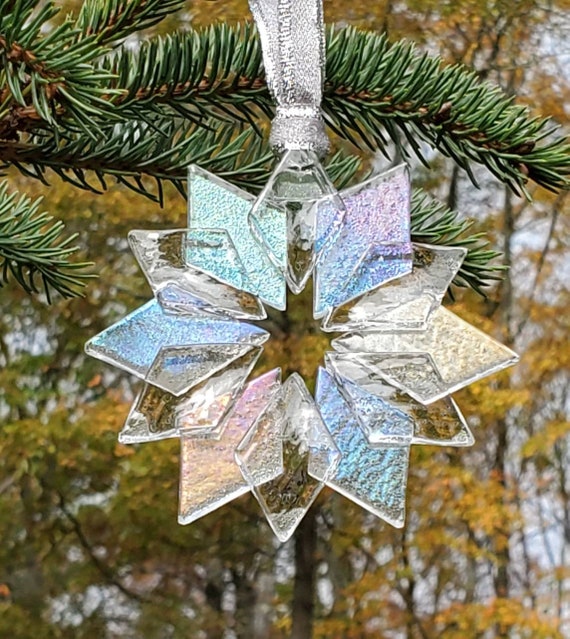The photograph showcases a Christmas tree ornament shaped like a snowflake, hanging from a silver ribbon. The ornament, made of both clear and colored semi-transparent diamond shapes, features small gaps in the center and exudes a frosty, metallic sheen. The topmost diamond, through which the ribbon is threaded, appears pristine and clear. Moving outward from the center, diamonds of various colors form the intricate snowflake pattern: teal on the top left, purple on the top right, blue on the left, gold on the right, peach on the bottom left, and light blue on the bottom right. The entire ornament glistens, mimicking the appearance of ice, though it is likely glass or plastic.

In the upper left corner of the image, delicate, thin green needles from a pine branch extend into the frame. The background reveals a serene outdoor setting with tall brown trees displaying an array of yellow and green leaves. Through the branches, a light blue sky dotted with white clouds is visible. The scene is framed within a rectangular photograph, encapsulating the enchanting contrast of the delicate ornament against the natural forest landscape.